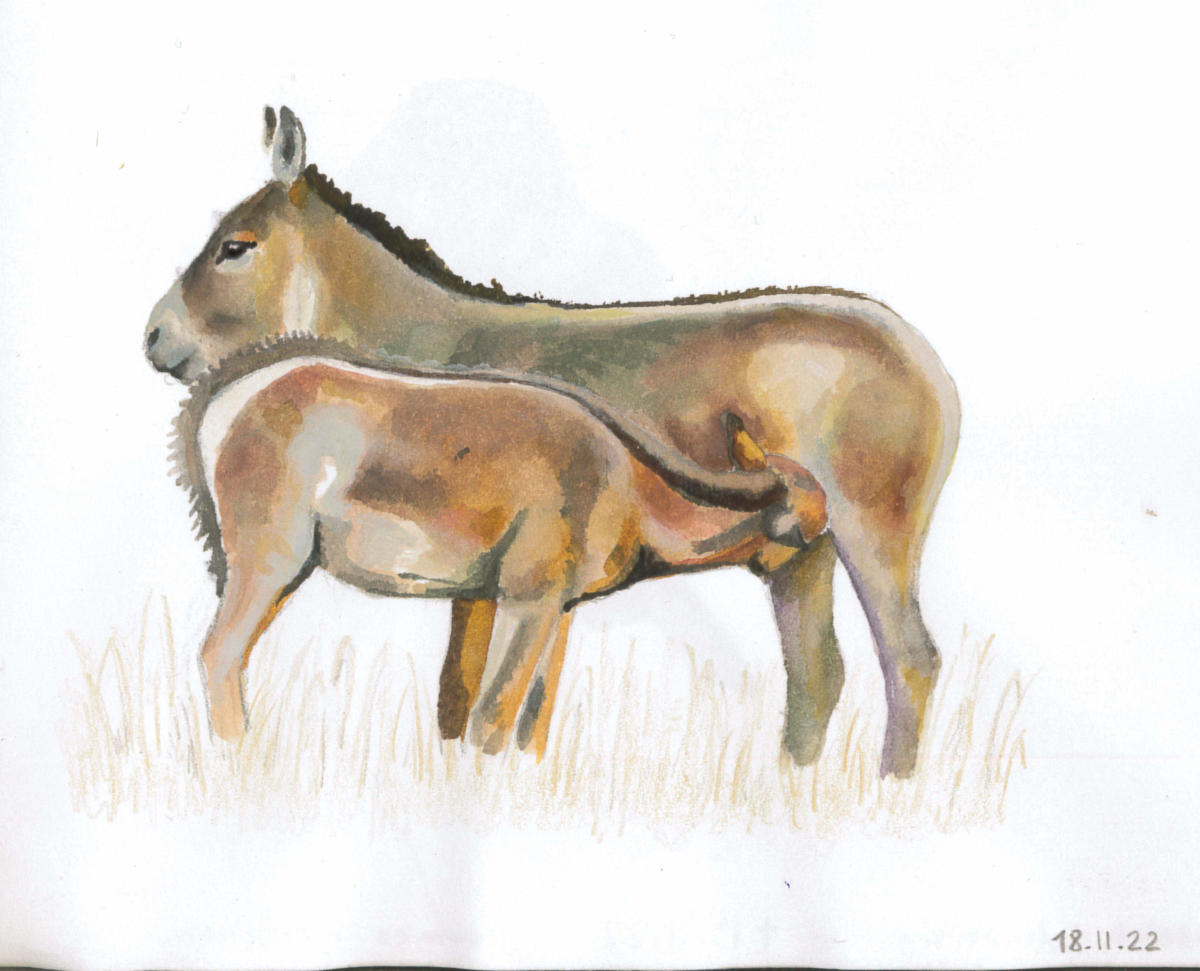The image is a watercolor painting with a blend of realistic and abstract elements, depicting a mother donkey and her nursing foal. The mother donkey, rendered in shades of brown and grey, stands facing left in a side profile. In contrast, the smaller donkey faces right, though its face is obscured as it suckles from its mother, showcasing a mix of reddish browns and tans. A dark brown line of hair runs from the top of the foal's head down its back. The background is stark white, with light brown patches of grass subtly shaded around the donkeys' legs. The painting is dated 18.11.22 in pencil at the bottom right corner.